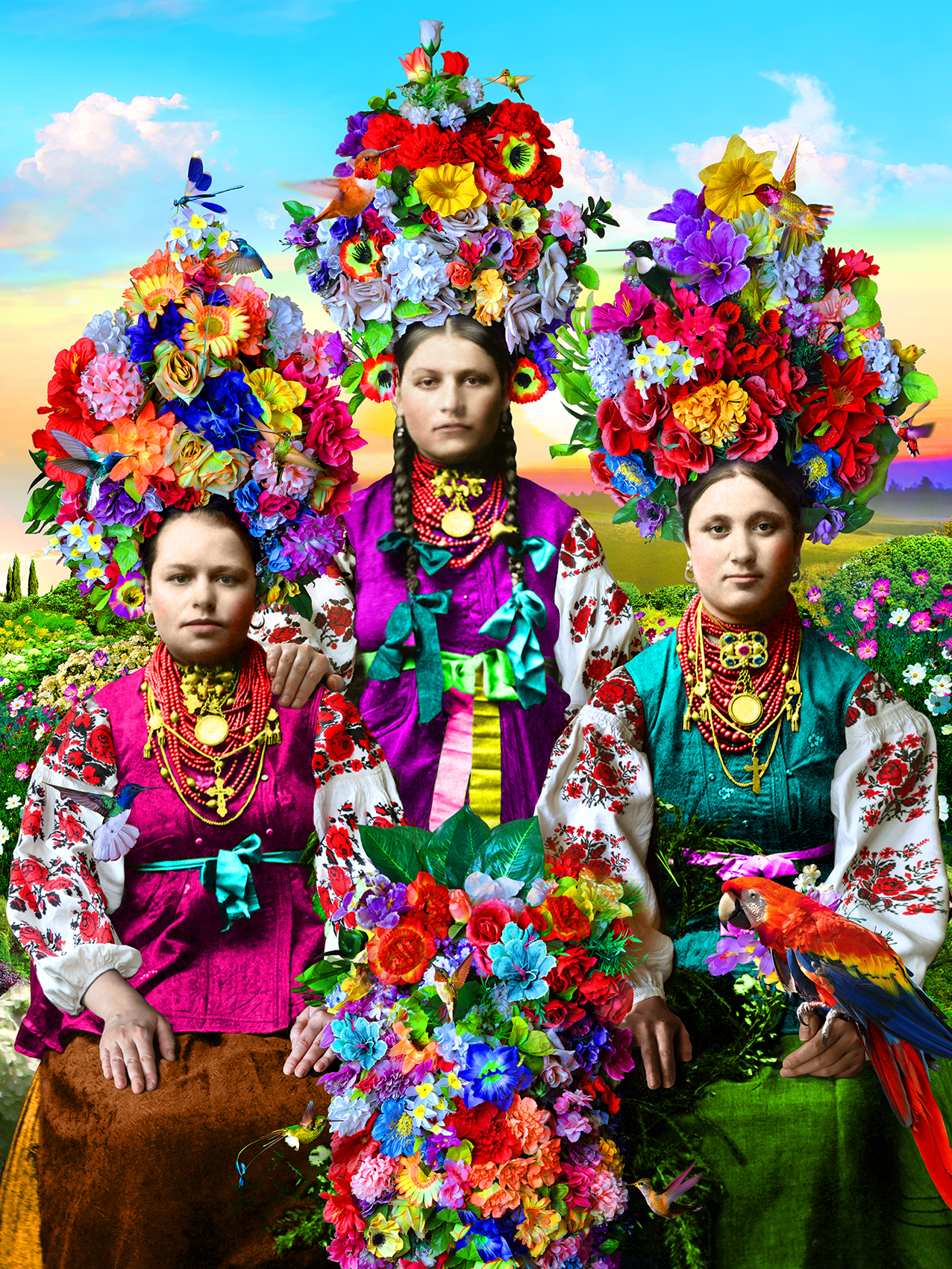The painting depicts three vibrantly dressed Native American women adorned in traditional festival or holiday attire, highlighting their cultural heritage. The women wear colorful, towering floral hats decorated with a myriad of flowers in hues of red, purple, blue, pink, and orange. Each woman is uniquely dressed: the left figure, possibly seated, wears a long brown skirt and a pink top with floral arm sections, complemented by a golden necklace with a cross. The central figure, identifiable by her two ponytail braids with blue ribbons, is dressed in a predominantly purple dress with green and yellow accents and a similar floral hat. The right figure, dressed in an aquamarine blue blouse and a grassy green skirt, also sports a decorative floral hat and has a bird resting on her hand. In front of them lies a colorful floral design that could be a bouquet or part of a dress. Their ensembles are completed with assorted beads, ribbons, and intricate prints, set against a backdrop of a blue sky with white clouds and hints of yellow. The image captures the essence of their vibrant traditions through the detailed and colorful representation of their attire and accessories.